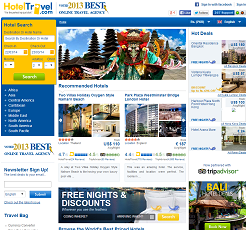This image is a website screenshot from "HotelTravel.com," dating back to 2013. The website features a partially legible banner proclaiming its accolades, although the full message is obscured due to fuzziness in that section. At the forefront, there's a prominently displayed hotel search form set against a yellow background. This form enables users to input their travel dates, the number of people, and the number of rooms required, culminating in a noticeable green search button.

Beneath the search form, several recommended hotels are showcased with accompanying images. Each hotel listing provides a star rating, pricing details, and additional markers, indicating various features or offers. Notably, prices are displayed in British pounds, suggesting the site's relevance to countries using this currency.

Adjacent to the hotel listings, there is a newsletter sign-up box where users can enter their email address. This section is highlighted with a blue "Submit" button, encouraging visitors to subscribe. Furthermore, an advertisement banner is visible, promoting "free nights and discounts," with an accompanying field to input information and a search function to explore these offers.